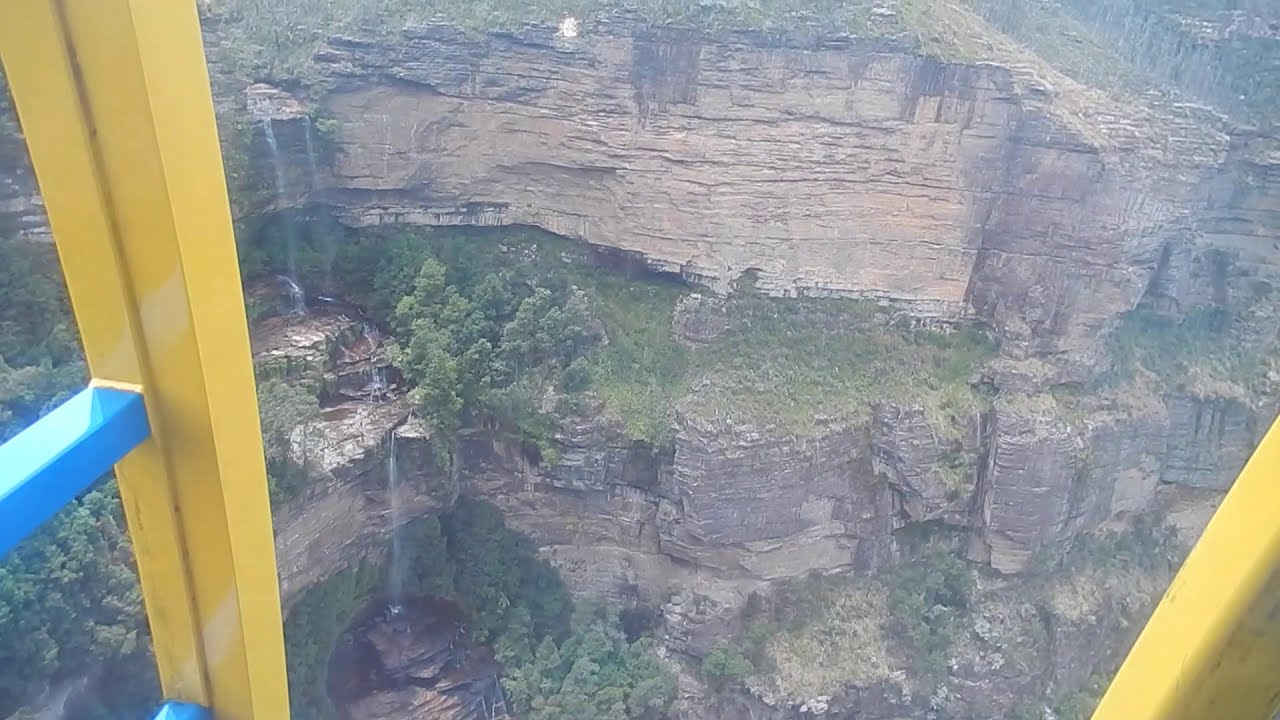The image showcases a high-angle view from an indoor facility, possibly a window of a tall structure. Prominently in the foreground is a yellow support beam with blue crisscrossed braces. This framing structure gives the impression of looking out from an elevated position onto a natural landscape. The scene outside is a rugged cliff divided into three sections, characterized by dark brown rocky walls, interspersed with patches of thin grass. On the left-hand side of the middle section of the cliff, there are large trees and a slender waterfall cascading down. The entire scene is bathed in natural daytime light, highlighting colors such as yellow, blue, green, tan, brown, and black. The focus remains on the contrast between the structured, metallic indoor setting and the untouched natural beauty of the cliffs and waterfall below.